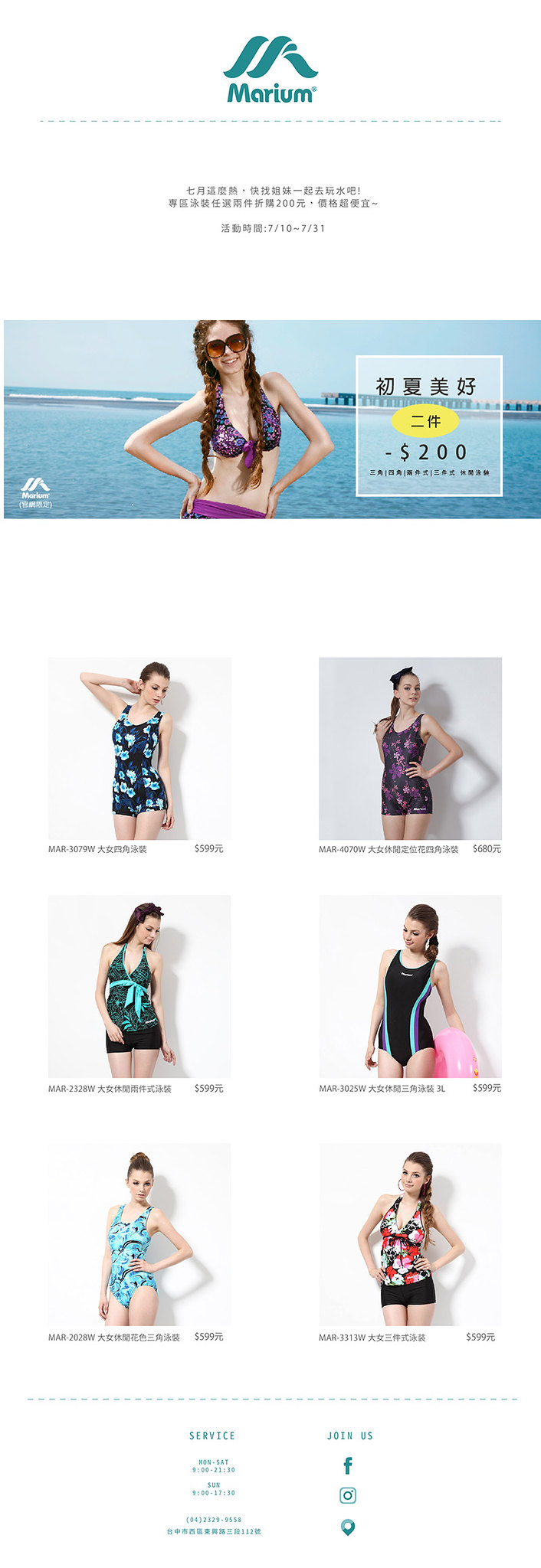This advertisement features a website branded as "Merriam," highlighted by a teal logo resembling two ocean wave arches above the name. Below the logo is text in an East Asian language, surrounding a primary photograph of a woman with dark brown, waist-length braided hair, wearing a purple and blue bikini. The woman, who has large sunglasses on and is smiling at the camera, stands in front of a picturesque ocean backdrop with a pier in the distance. To the right of this main image is a text box stating "$200 off," while below it, a series of six smaller images showcase the same model in a variety of one-piece swimsuits, presented against a white background. The designs of these swimsuits vary, including different colors like purple, blue with light blue flowers, and black with aqua stripes. At the bottom of the advertisement, there are social media links, though the smaller size and color make them difficult to discern clearly.